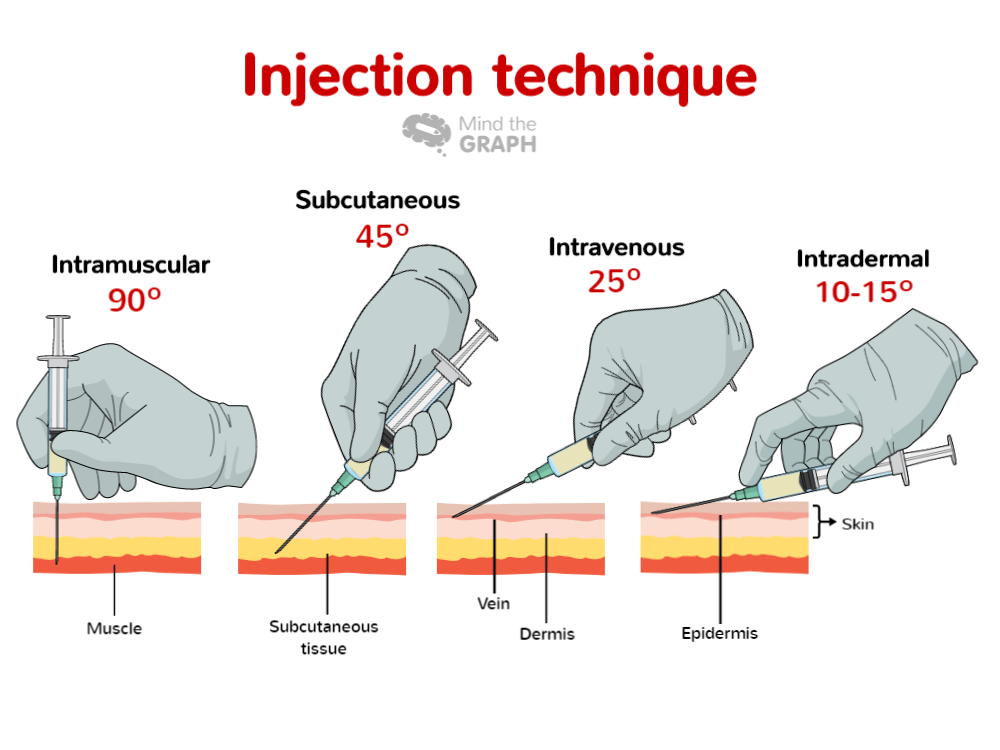The image is an illustrative guide from medical personnel on injection techniques, prominently labeled "Injection Technique" at the top in red text, with a gray "Mind the Graph" logo just below. It systematically demonstrates four types of injections, each depicted with a gloved hand inserting a needle into different layers of tissue. The first illustration shows a 90-degree angle needle insertion into the muscle, labeled "Intramuscular." The second illustrates a 45-degree angle insertion into the subcutaneous tissue, labeled "Subcutaneous." The third displays a 25-degree angle insertion into a vein and the dermis, labeled "Intravenous." The fourth image depicts a 10- to 15-degree angle insertion into the epidermis, labeled "Intradermal." The tissue layers are represented by colored layers in shades of pink, beige, yellow, and red. All hands are shown wearing gray medical gloves and each needle is angled appropriately for the respective injection technique.